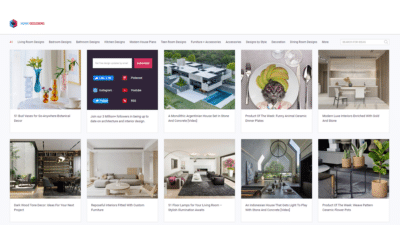This image is a screenshot of a web page featuring a header and a grid of photos. The image quality is poor, making the fonts and details difficult to discern. At the very top against a white background on the left side, there is an unreadable company name and logo. The company name is a single word with one-third of the letters in light blue and the other two-thirds in a pinkish-red color. The logo resembles a cube divided into the same blue and pinkish-red colors but is not clear enough to be read.

Below the logo, a header menu with a very light gray background and several gray-font items is visible, though none of the text is legible due to the small and blurry print. Dominating the rest of the web page are two rows of photos, each row containing five images except for the top row, which has a search box in the second position from the left. The search box has a black background and a white rectangle within it, likely serving as the search field. A red button, probably the search button, and six unreadable items are also present.

The upper left photo shows a table adorned with several vases and positioned near a window. The far-right image in the top row appears to be of a large dining room, although it is unclear whether it is a photo or a drawing. The bottom row contains five photos predominantly featuring interiors with very light, off-white color schemes. The lower right corner image seems to depict an outdoor terrace with clay pots housing green plants and possibly a ledge in the background.